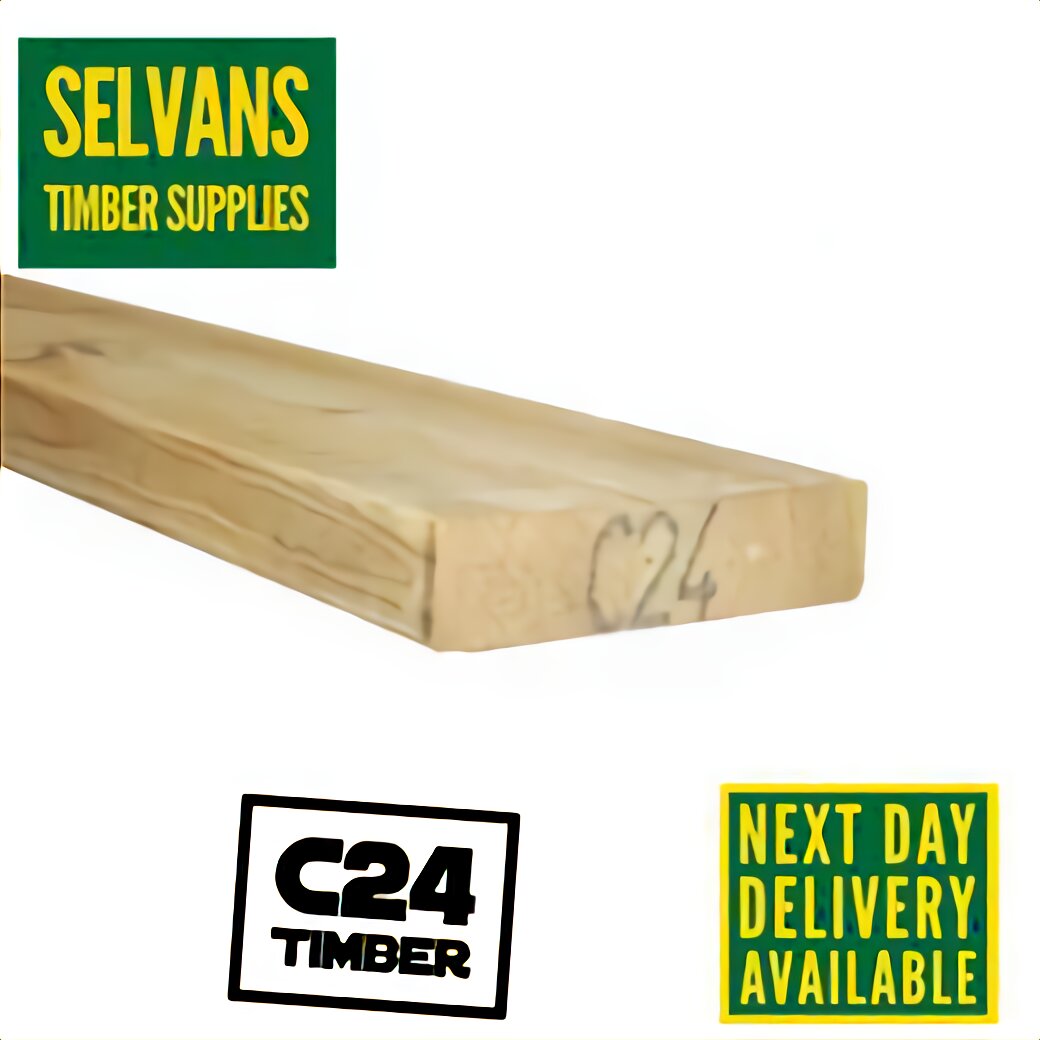The image features a screenshot with a clean white background, prominently displaying multiple visual elements related to a timber supplies business. At the center lies a wooden slab adorned with the inscription 'C24' in brown lettering, indicative of the timber grade. Above this slab, there's a green square framed by a yellow outline, containing a message in the same yellow hue that declares "Next Day Delivery Available." Scattered across this square are a few small blue dots, adding a distinct but subtle pattern.

Adjacent to these elements is a black square bearing the text 'C24 Timber.' In this block, the 'C24' text is slightly larger than the word 'Timber,' highlighting the specific type of timber. Moreover, the business name, 'Selvin's Timber Supplies,' is prominently featured in yellow text, with 'Selvin's' in a much larger font size—approximately three times larger—than the accompanying 'Timber Supplies,' ensuring the brand name stands out clearly.

Overall, the alignment and color scheme of the various shapes and texts create a visually coherent and enticing advertisement focusing on quality timber and swift delivery service.